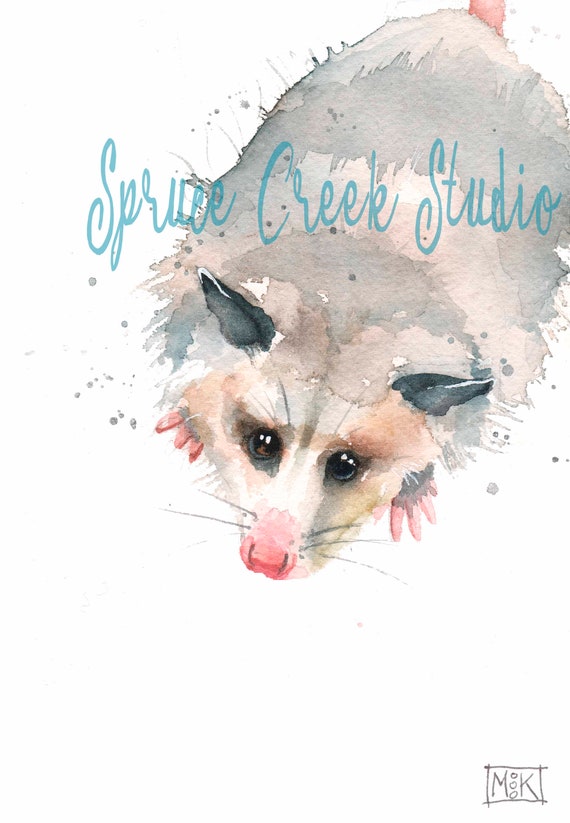This image depicts a detailed watercolor painting of a gray and white opossum lying flat against a white background. The viewer is given an overhead perspective, allowing a clear view of the opossum's body and head. The opossum has a cute face with a pink nose and black eyes, its distinct black pointed ears standing upright above its eyes. The painting also captures its delicate pink and black-tipped claws on its feet, positioned at either side of its body.

The opossum has a light gray body with subtle white blending, characteristic of watercolor art. Positioned across the opossum's body in teal cursive text is the watermark "Spruce Creek Studio", serving as an elegant, identifiable mark of the artist's studio. Furthermore, at the bottom right-hand corner of the image, the artist's initials "MK" are handwritten within a small box, adding a personalized touch to the artwork.